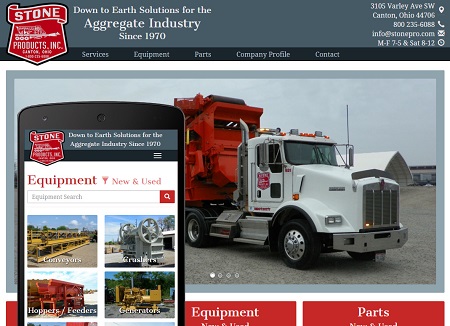This image is a screenshot from a website related to either equipment rental or sales, though the specific focus is unclear. The company's name is Stone, prominently featured with its logo in the upper left-hand corner. The logo is red with white text, and it overlays a dark gray header bar that also has white text.

Beneath the header is a standard black menu strip with white text displaying the categories: Services, Equipment, Parts, Company Profile, and Contact. On the far right-hand side of the header, there is the company's address and contact information.

Immediately below the menu, there is a large, striking image of a tractor-trailer transporting equipment. Superimposed on this image is the depiction of a smartphone screen, showcasing a mobile version of the company's website. This suggests that the website is accessible and fully functional on mobile devices, allowing users to easily contact the company or browse their services.